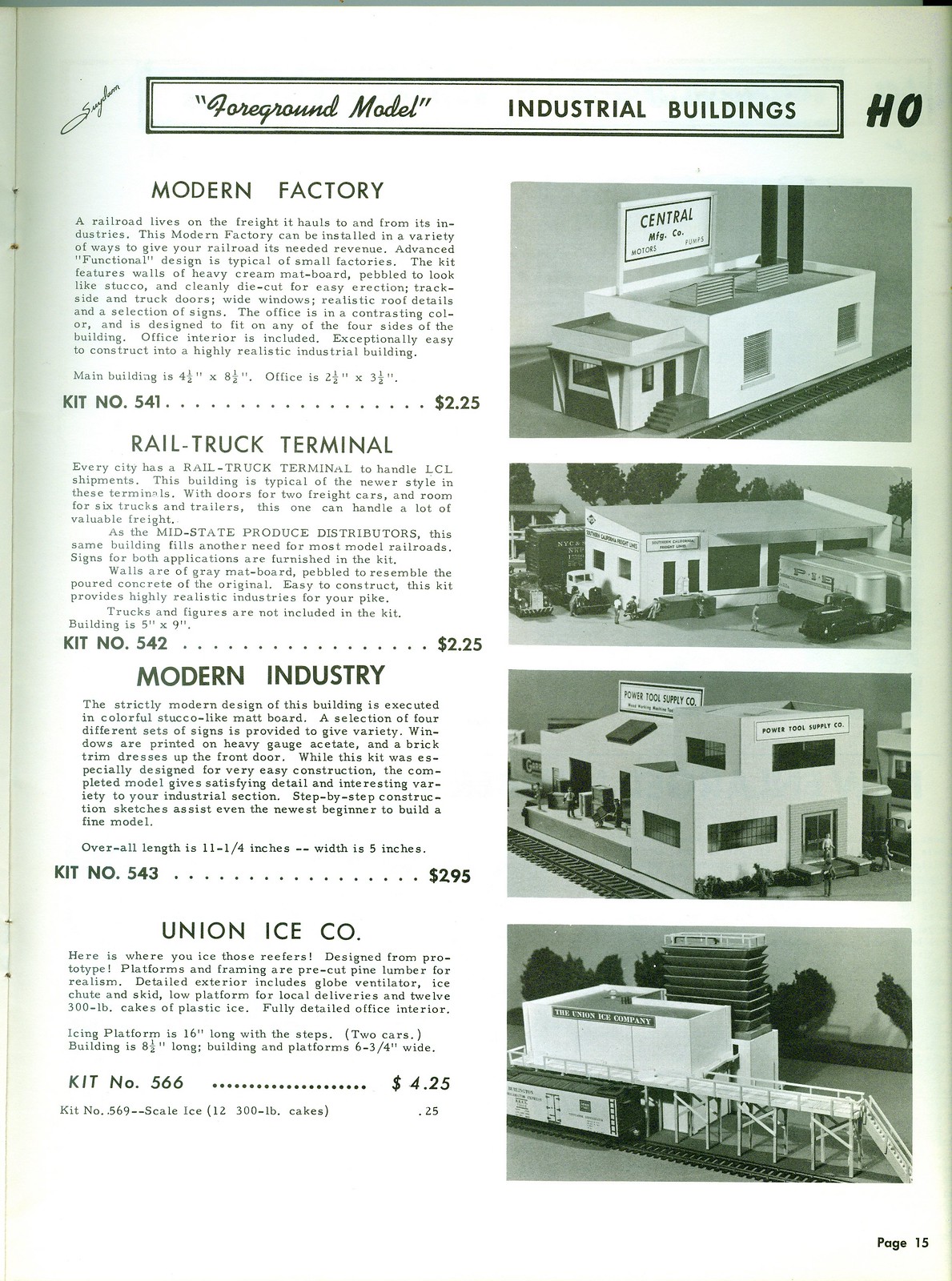The image is a detailed page from an old magazine, specifically page 15, showcasing various diorama-like models under the title "Foreground Model Industrial Buildings." At the top, "Foreground Model" is written in cursive quotes, while "Industrial Buildings" is in all caps. The page features images of model buildings on the right with corresponding descriptions, kit numbers, and prices on the left. 

The first model labeled "Modern Factory," kit number 541, priced at $2.25, includes detailed text describing its advanced functional design, realistic roof details, wide windows, and adaptability for trackside installation. The factory can be installed in various ways to provide immediate revenue for a model railroad.

Below, "Rail Truck Terminal," kit number 542, also priced at $2.25, is showcased with a vertical structure and a slanted roof. 

Next, "Modern Industry," kit number 543, priced at $2.95, is a two-floor building highlighted for its realistic features.

Finally, at the bottom, "Union Ice Co.," kit number 566, priced at $4.25, is another two-floor building.

Each model is meticulously described and accompanied by realistic images to enhance the appeal to model railroad enthusiasts.